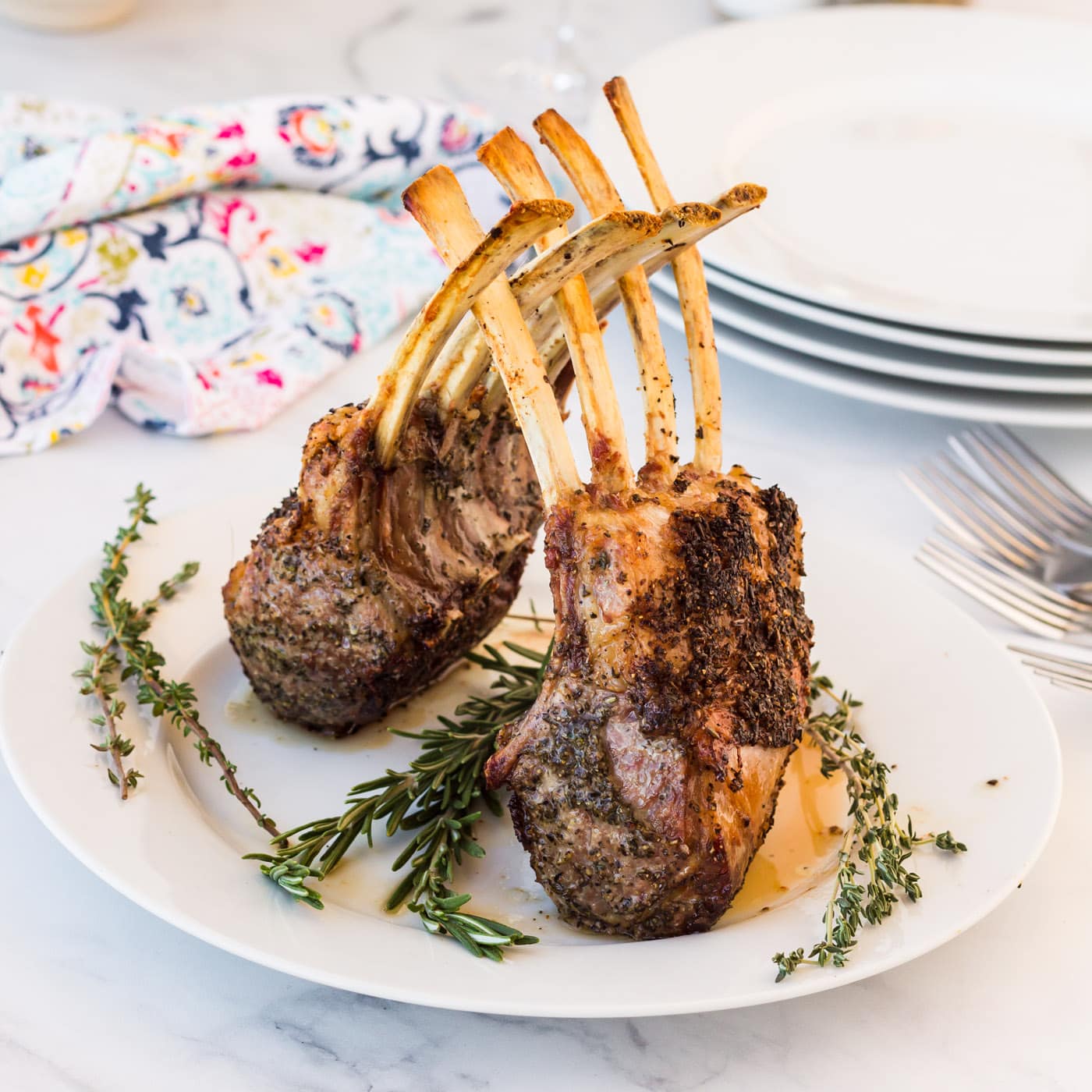In this staged, color photograph taken indoors with artificial lighting, a vertically rectangular image captures a delectable culinary presentation on a white marble surface streaked with subtle black and gray highlights. At the center stands a plain white plate showcasing two well-cooked racks of ribs, their bones artistically intertwined to form an engaging visual. Garnishing the plate are fresh sprigs of rosemary or thyme, adding a delicate touch of greenery to the browned, savory meat. To the right of the plate, a stack of four plain white plates is neatly presented, alongside four polished silver forks arranged in a line. In the upper left-hand corner, a vibrant cloth napkin with patterns of blue, pink, and yellow adds a splash of color to the otherwise elegant and minimalistic setting, giving the impression of a thoughtfully curated meal ready to be enjoyed.